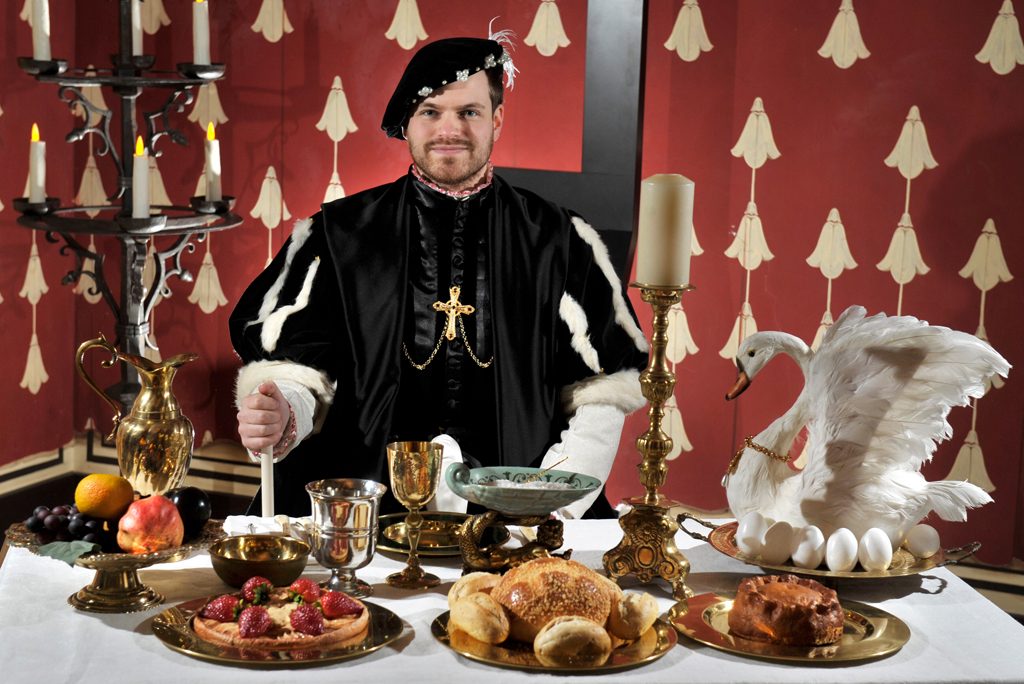This photograph captures an indoor scene reminiscent of medieval times, featuring a male performer or cosplayer dressed in elaborate period attire. Standing from the waist up behind a lavishly set dinner table, the individual sports a black outfit with distinctive poofy arm sections extending from the shoulder to the elbow, under which white sleeves are visible. A trimmed beard and a black hat with white designs around its circumference complete his outfit, along with a golden cross hanging on his chest, suspended by two chains that disappear beneath his outer shirt.

The dining table in front of him is adorned with a white tablecloth and an array of medieval-style food displayed on golden platters. Notable among the spread are bread rolls, a pie topped with strawberries, a fruit bowl, and several ornate wine chalices. The table also features a variety of decorative elements, including two candle holders: a particularly elaborate one on the left holding several candles, and a simpler yet striking one on the right. Amongst this feast, an eye-catching prop is a life-sized, inanimate bird—likely a swan or goose—adorned with a gold chain and surrounded by bird eggs, resting majestically on another golden platter.

The backdrop of the scene emphasizes the medieval ambiance, with deep red wallpaper decorated in a gold repeating pattern, adding to the historical feel. The overall setting is well-illuminated but within an indoor context, making it difficult to ascertain the time of day. The gentleman stands facing the camera, with one arm extended and the other resting at his side, poised amidst an impressive display of replicated medieval opulence.